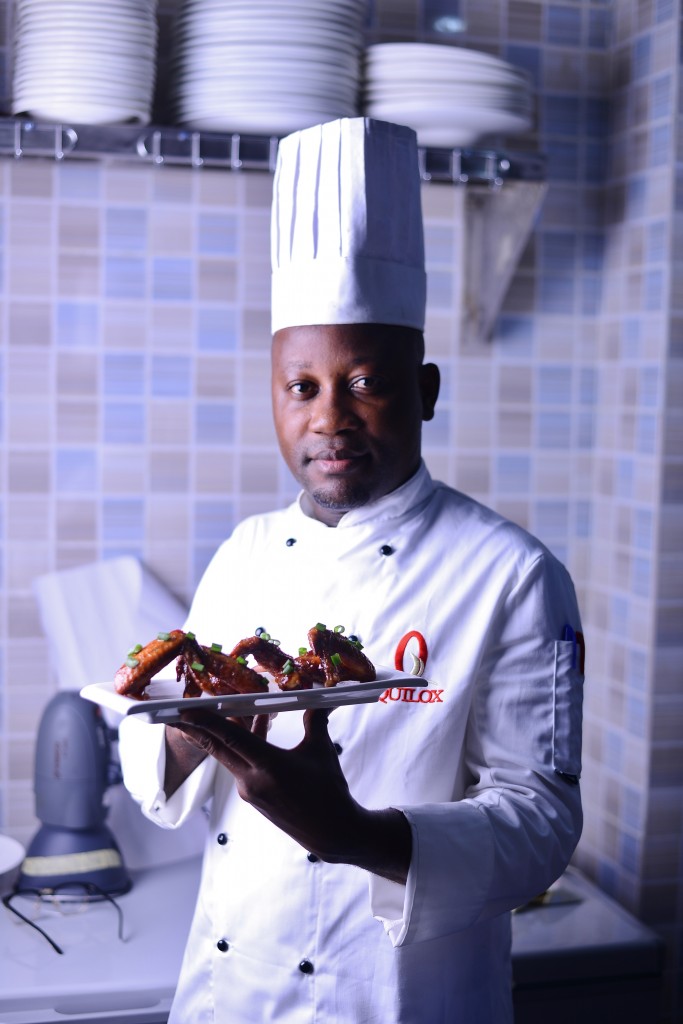This is a detailed vertical rectangular photograph of a black chef proudly presenting a plate of food in a kitchen. The chef, dressed in a traditional white chef’s coat featuring a red logo, and a white chef’s hat, holds the plate with his left hand while steadying it with his right. The food appears to be barbecued chicken wings, fried to a rich brown and artfully arranged with a sprinkling of chopped parsley.

The background is a mosaic of small tiles in shades of light blue, tan, and brown, adding a decorative touch to the scene. Above the chef are shelves holding neatly stacked plates, and behind him is a counter cluttered with kitchen essentials, possibly including dishes and a mixer. The chef’s demeanor exudes pride as he showcases his culinary creation in this vibrant kitchen setting.